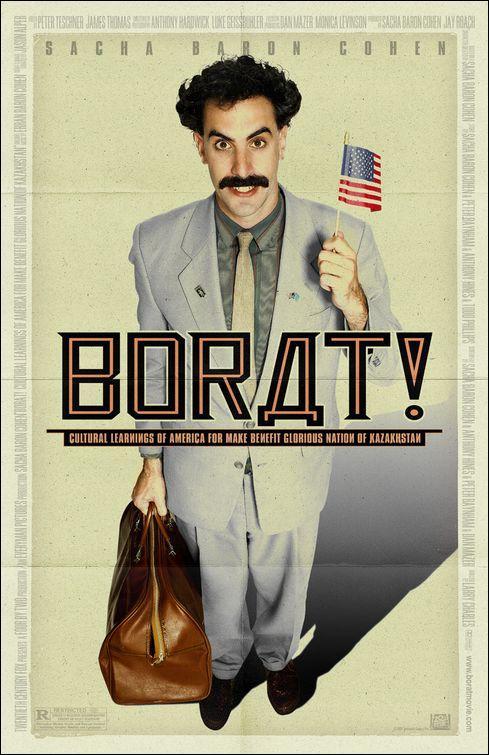This promotional poster for the movie "Borat" features a large rectangular design with an off-white, yellow-beige background. Surrounding the edges are names and movie details in a light font that blends with the background, making them hard to read. At the very top, it prominently displays the name "Sacha Baron Cohen." Below, Cohen appears as his character Borat, dressed in a gray suit, gray pants, brown shoes, a tan tie, and an off-green shirt. He sports a large mustache, bushy eyebrows, messy hair, and a slightly manic expression. In his left hand, he proudly holds a small American flag, while his right hand carries a brown leather suitcase. His shadow is visible behind him, adding depth to the poster. Centered in bold text is the movie title: "Borat! Cultural Learnings of America for Make Benefit Glorious Nation of Kazakhstan."